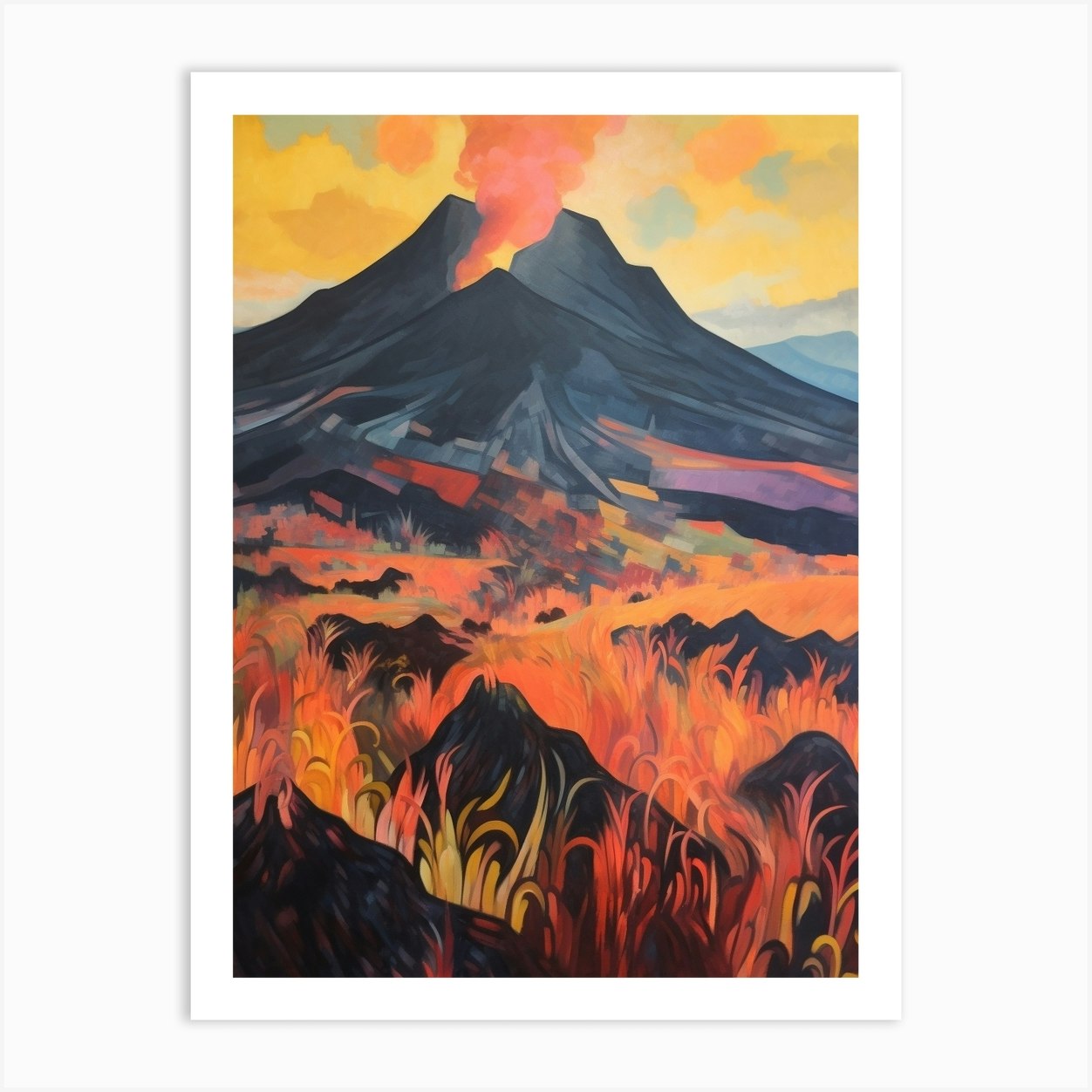This is a vivid oil painting, possibly computer-enhanced, depicting an active volcanic eruption at sunset. The volcano dominates the scene with its imposing, black and gray mountain, crowned by a large chasm at the top that emits a plume of orange and red fumes. Fiery lava flows cascade down its slopes, interspersed with bursts of red and yellow flames that engulf the rocky outcroppings in the foreground. The sky is ablaze with hues of yellow, orange, pink, and red, enhancing the intensity of the eruption. At the volcano's base, a field features a mix of black lava rocks and multicolored, flame-like grass, creating a striking contrast between the earth's raw power and the resilient flora sprouting amidst the remnants of past eruptions.